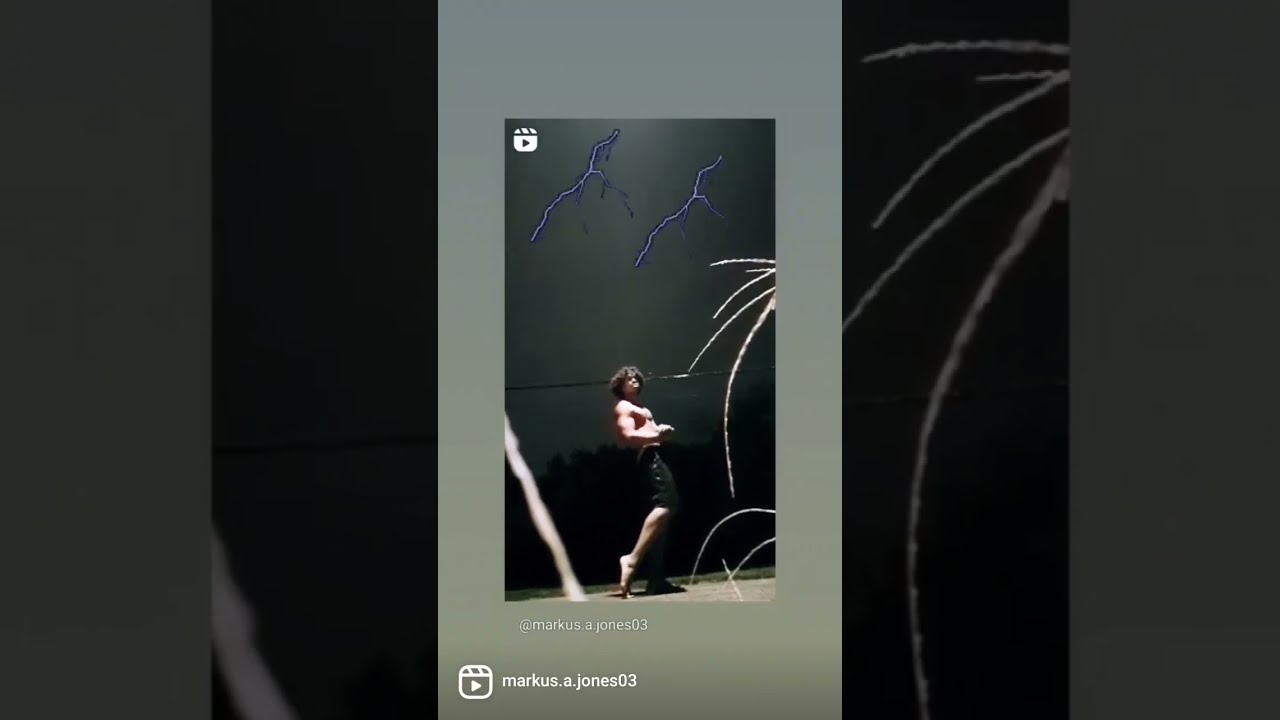The image is an advertisement for a video featuring a shirtless man with long, dark brown curly hair that falls over his ears. He stands in the center of the image, clad in black shorts that reach his knees. The man striking a bodybuilding pose, facing towards the right, with his right arm flexed and his right calf accentuated by having his toes touching the ground while his heel points directly upwards. His left foot, which is under a shadow, is flat on the ground. Above the man, there are stylized purple lightning strikes and white streaking lines, giving the illusion of electricity or energy, against a backdrop of a dark gray wall that fades to a deeper shade towards the bottom. 

The focus of light is directly on the man, emphasizing his muscular physique. Below him, the text "@marcus.a.jones03" is displayed, accompanied by a play button that repeats the handle "marcus.a.jones03." In the upper corner, another play button is visible. The image is framed within a gray box, and on either side are tinted, zoomed-in sections of the main image: the right side shows a close-up of the white streaking lines, while the left side features an angular segment of a white bar. Overall, the image exudes a dark yet dynamic atmosphere, centered around the powerful and energetic depiction of the man.